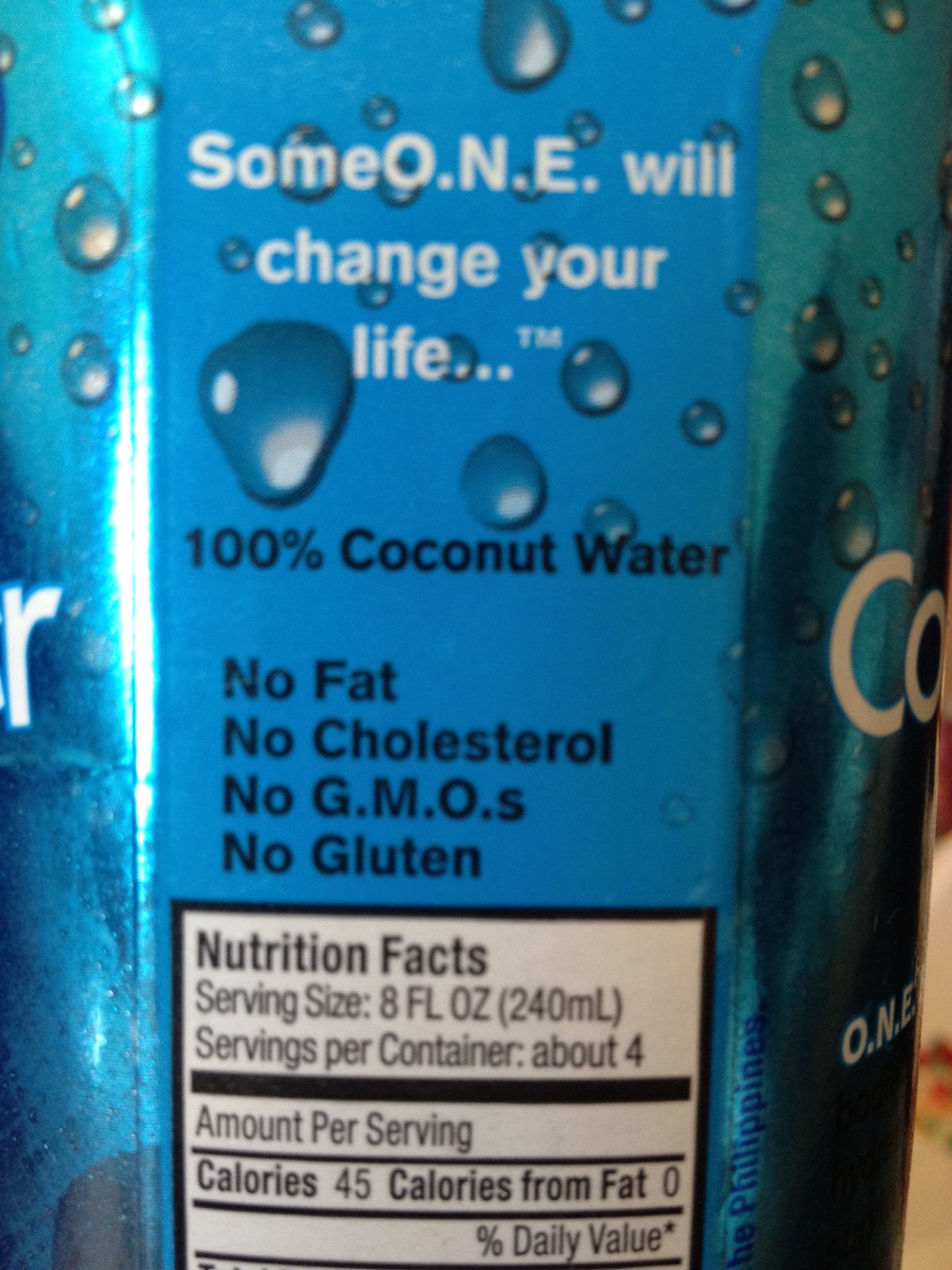A close-up image of a sleek and modern coconut water bottle, primarily blue in color. The central panel of the bottle features a deep blue background with white text that declares, "Someone will change your life...™". Below this inspirational statement, black text lists several health benefits of the drink: "100% coconut water, no fat, no cholesterol, no GMOs, and no gluten." To the sides of this panel, the bottle showcases metallic teal-aqua hues, embellished with design elements that mimic droplets of water, giving the illusion that the bottle is refreshingly cold and perspiring. A white box with a black border provides the nutrition facts, detailing a serving size of 8 fluid ounces (240 ml) with approximately 4 servings per container. Each serving contains 45 calories, with 0 calories from fat, though the full list of daily values is not fully visible in the image. The combination of sleek colors and detailed information emphasizes both the modern appeal and health-conscious benefits of the product.